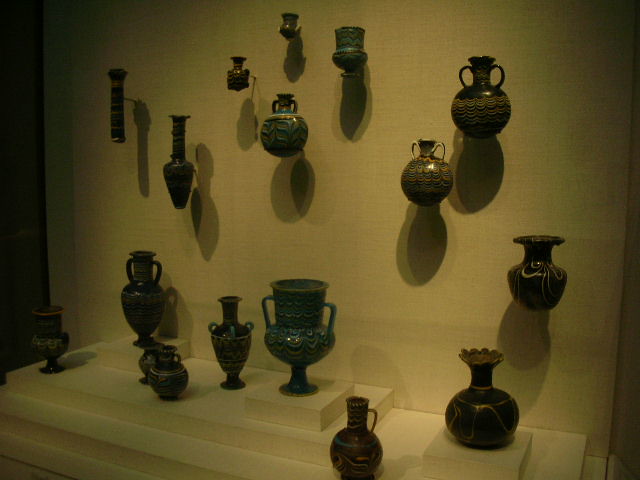This is a photograph of an art museum display featuring a rich assortment of chalices, vases, and urns. Arranged against a light tan wall and on a white multi-tiered stand with varying levels, the pieces exhibit an intriguing variety of shapes and designs. The wall on the right side angles slightly towards the camera, with vases and urns meticulously positioned throughout.

On the left side, a tall, slender vase with a long neck that bulges out towards the base stands prominently. Nearby, two small, scarcely visible vases are placed above a large, round urn with two side handles. A short, wide vase with a uniform width throughout is also noticeable in the display. Moving down and to the left, a large bowl-shaped vase features two prominent handles looping from the body to the top. Right above it, an identical design is presented in a dark brown color.

In the lower right corner of the wall arrangement, an impressive vase features a broad base, wide neck, and flaring top with no handles. On the white stand below, the varied heights of the vases create a dynamic visual effect. To the far left, a tall vase with a slender neck and small base stands out, flanked by a vase with an intricate design of three handles and a long, slender body. Another notable piece is a large urn with a substantial neck and bulbous base tapering to a narrower bottom.

Among other highlights, a vase with a big bulb and thin neck, fanning out at the top like a flower, adds a remarkable touch to the collection. From dark brown urns with intricate patterns to large vessels with wide openings, this exhibit showcases an exquisite variety of pottery, illustrating both artistic diversity and craftsmanship.